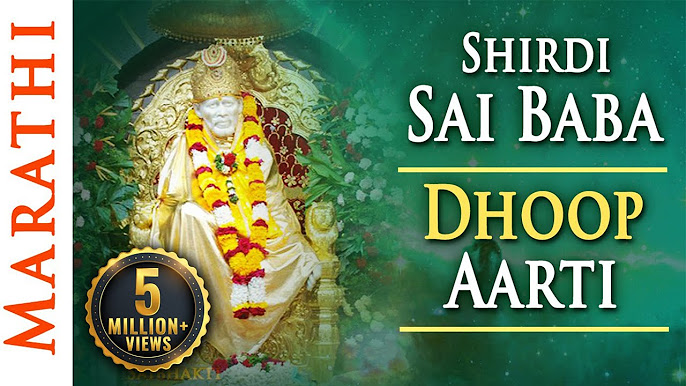The image is an advertisement that prominently features a seated statue of Shirdi Sai Baba, gilded in gold. The statue, possessing a dignified and serene presence, wears a golden crown and gold robes, and is adorned with a long lei made from red, white, and yellow flowers. Shirdi Sai Baba's visage is completely white, suggesting either a statue or a face painted in pristine white, and he is seated on an ornate gold throne surrounded by a vibrant arrangement of red and white flowers with green leaves. The backdrop is a shimmering green, enhancing the statue's celestial appearance.

Text overlays enhance the advertisement's visual appeal; "Shirdi Sai Baba" appears in white text on the right side of the image. Below it, separated by two yellow bars, the words "Dhoop Aarti" are displayed, with "Dhoop" in yellow and "Aarti" in white. Additionally, a word spelled "M-A-R-A-T-H-I" is written vertically in red text on the far left side, requiring viewers to tilt their heads to read it correctly. Completing the design, a badge positioned in the lower left-hand corner indicates the ad's popularity, stating "5 million views" within a black circle edged in gold.